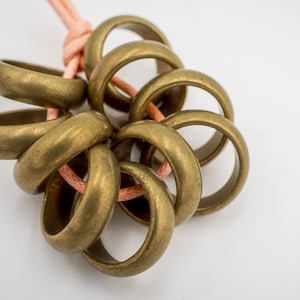The image features a close-up of a light pink rope hanging against a very pale blue or off-white background. At the bottom of this rope, there is a loop securing approximately nine gold rings, though some may appear tan or brown due to lighting or wear. The rings, which are overlapping each other, could be made of wood or plastic, and they have an aged, well-worn look. The positioning of the rope suggests it is tied or hanging from something above, with the rings clustered near the end. The simplicity of the composition highlights the intriguing collection of rings on the cord, evoking thoughts of wedding bands or vintage carousel ride tokens. The purpose of the arrangement remains unclear, adding a layer of curiosity to this otherwise minimalistic scene.